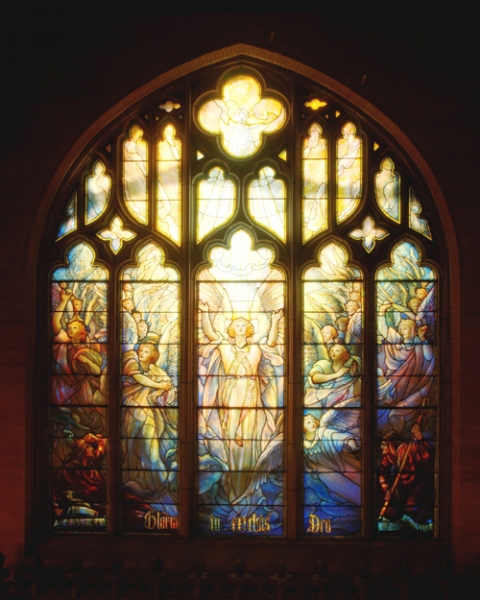This vertically aligned rectangular picture depicts a stunning stained glass window, characteristic of those often found in churches, featuring an arched top with intricate cutouts through which a radiant yellow light shines. Central to the composition is a larger, middle pane that showcases a golden and white angel, her arms raised and gaze directed upwards, illuminated by the light behind her. Surrounding the angel on either side are vertical rectangular sections with various outlines of people adorned in hues of blue, red, brown, and even green, probably representing religious figures. The bottom portion of the picture is notably dark, indicative of a dark brown wall likely positioned below the window, with a dark brown border framing the stained glass. This border arches upwards and terminates with a slight tip at the very top, capped by solid black color. No text or words are present in the image, and the scene is accented with additional crosses, including a prominent one at the top, further suggesting a religious setting. The background is dark, making the vibrant colors of yellow, orange, red, blue, light purple, and brown of the stained glass stand out sharply against it. All pictured figures face the viewer directly, enhancing the sense of solemnity and reverence conveyed by this captivating piece.